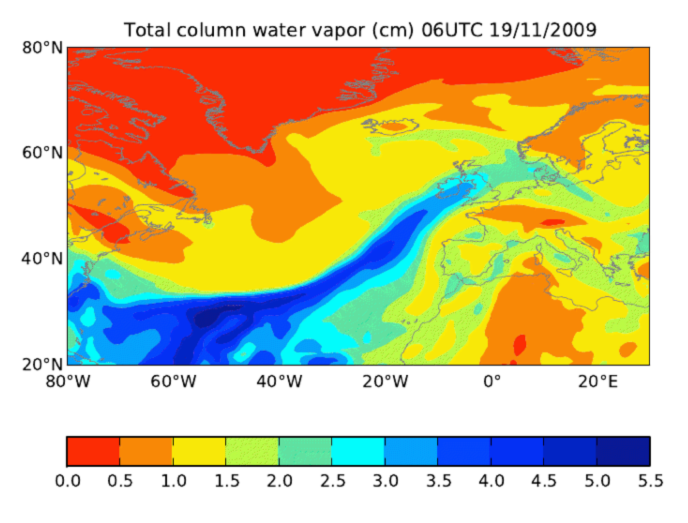The informational chart displays a detailed map titled "Total Column Water Vapor (CM), 06UTC 19-11-2009," marked in black text at the top. The map features a large area with various colors indicating different water vapor intensities. On the left side of the map, a vertical scale runs from 80 degrees north to 20 degrees north in 20-degree increments. Horizontally along the bottom, degree markers range from 80 degrees west to 20 degrees east, also in 20-degree increments, passing through 0 degrees. A vivid color gradient at the bottom of the map, transitioning from red to indigo, represents water vapor values from 0 to 5.5 centimeters. The map shows detailed color variations, including red at the top, transitioning through orange, yellow, green, and blue towards the bottom, highlighting different areas' water vapor concentrations.